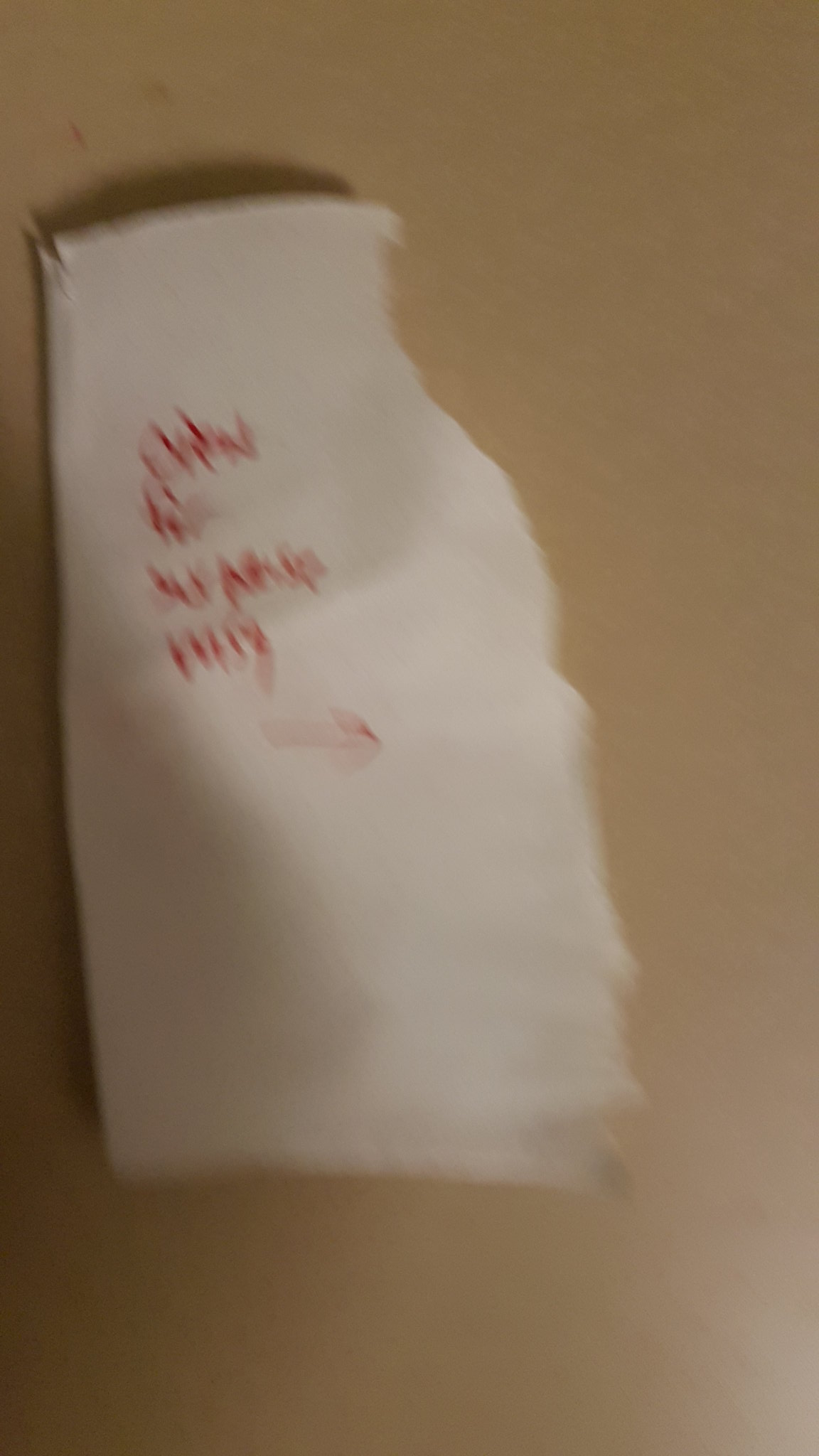This is an extremely blurry photograph of a torn piece of white paper lying on a flat surface, likely a countertop or floor with a light to dark brown hue. The roughly ripped paper features jagged edges, especially on the right side, while the left edge remains relatively straight. Written in red marker on the paper are four distinct lines of text, each word stacked below the previous one, but the blur obscures any attempt to decipher the letters. Below the fourth word, a thin red arrow points towards the right side of the image. The photograph suggests a darker area on the left side, hinting at a light source coming from the right. The overall scene feels disorganized and haphazard due to the condition of the paper and the photograph's poor quality.